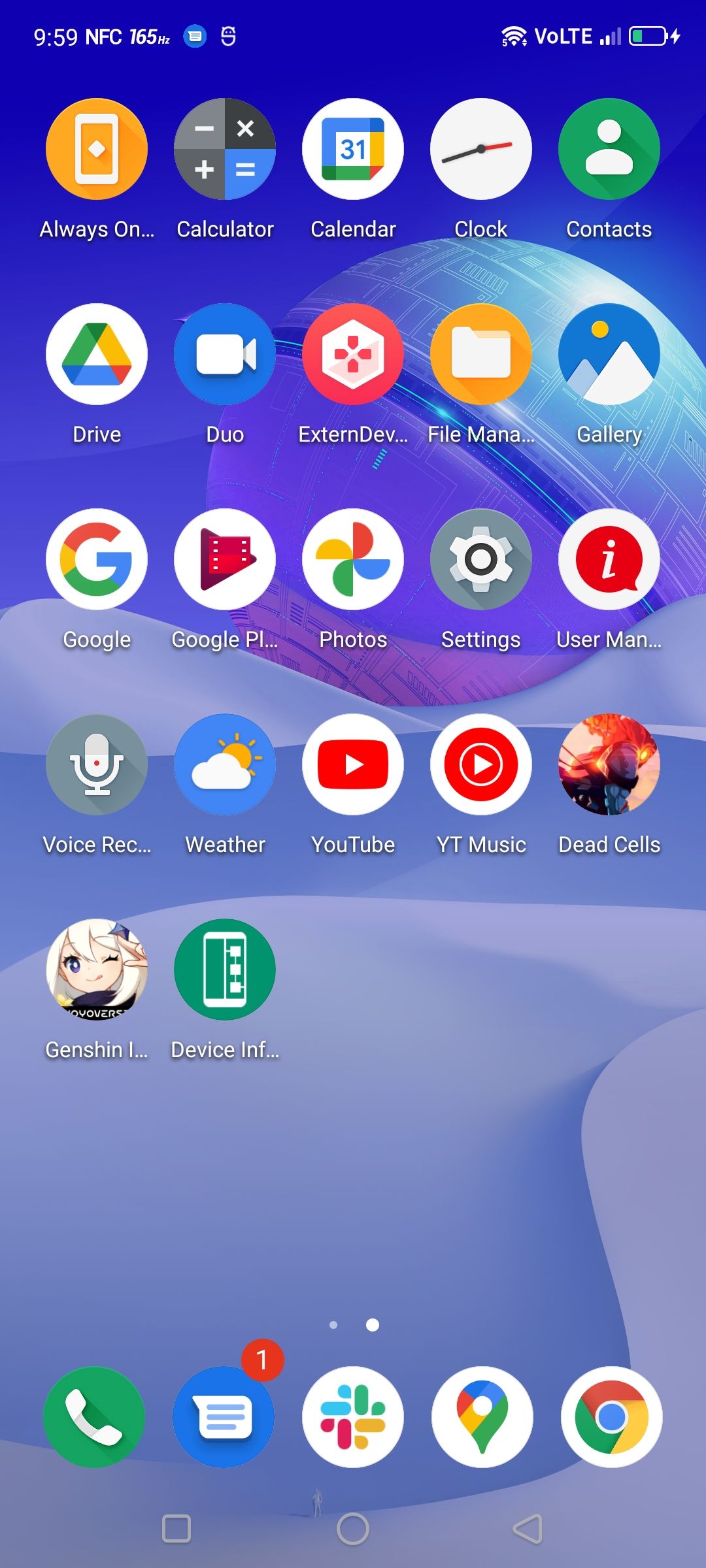The screenshot displays the home screen of an Android phone. The status bar at the top includes several indicators: on the left, "9:59" is displayed in white text, followed by "NFC 165 HD" and several symbols. On the right side, the indicators display Wi-Fi signal bars, "V-O-L-T-E," cellular signal strength with two out of four bars filled, and a battery icon. The battery icon shows the phone is charging, as evidenced by a lightning bolt next to it, and a green bar within the battery symbol indicating a charge level of approximately 30%.

The main background of the home screen features an abstract, predominantly bluish and slightly purplish and grayish image, possibly depicting a planet. The screen is populated with various app icons, including Drive, Google, Weather, YouTube, Dead Cells, Settings, Duo, Gallery, Contacts, Clock, Calendar, and Calculator. Some icons are not fully visible and are indicated by ellipses.